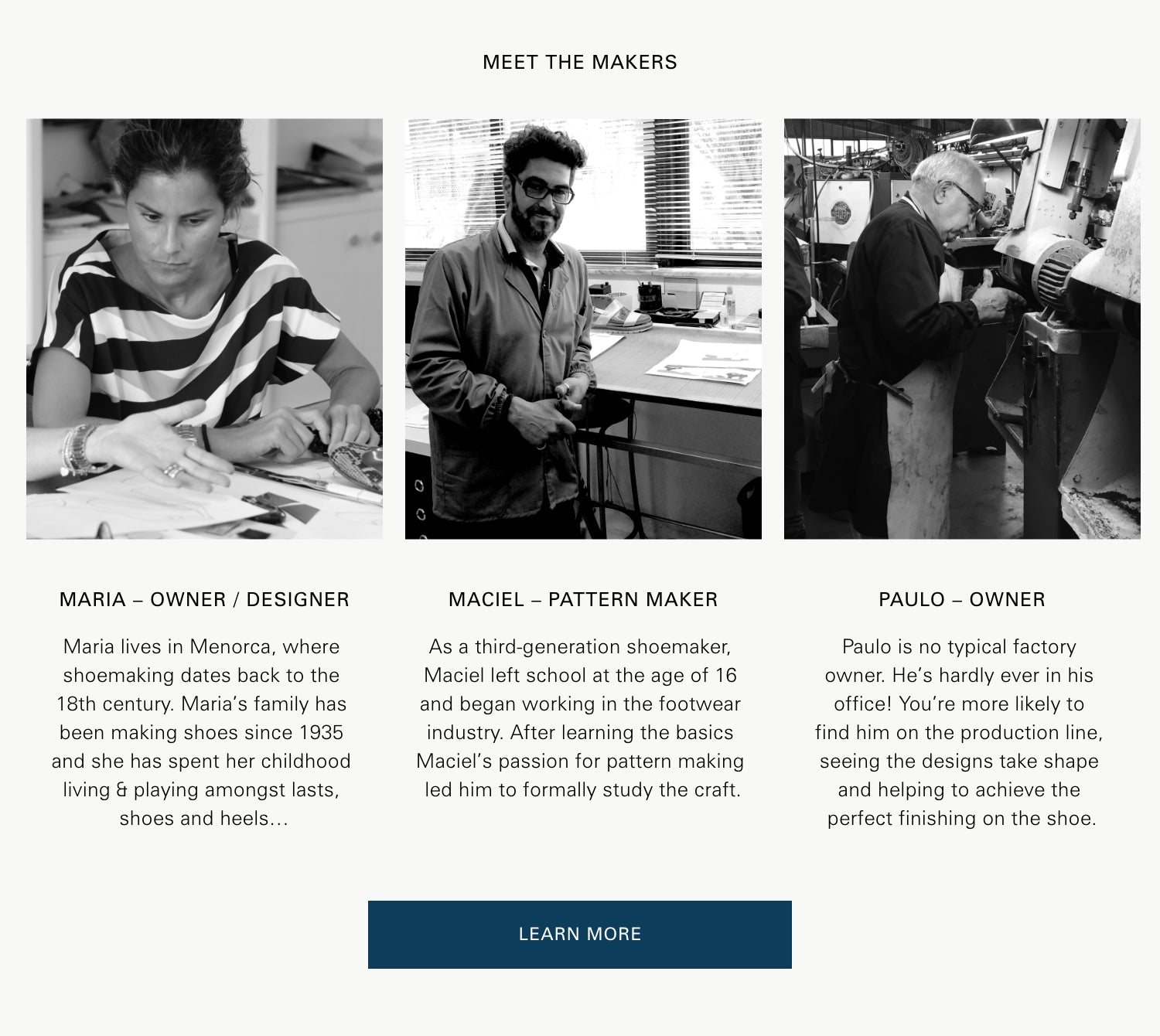This is a large square image with a light gray background and a small, all-caps black text title at the top that reads "MEET THE MAKERS." Across the center are three black-and-white photographs with small gaps between them, revealing the light gray background. 

On the left, the photo features a woman named Maria, who is the owner and designer. She is wearing a striped short-sleeved top with her hair pulled back, focusing on some papers on her desk. There's a second hand in the frame, pointing at something she is examining closely. Below her picture, there's a biographical paragraph detailing her background.

In the middle photo is a man named Maciel, a pattern maker. He stands in front of a drafting table near some sunlight-filled windows, dressed in a light to dark jacket over an open collared shirt. He has tall curly hair on top, short sides, a beard, a mustache, and wears black glasses. He is smiling at the camera with his hands clasped near his stomach. His biographical paragraph is below his image.

On the right, the third photo shows an older man named Paolo, who is the owner. Wearing glasses and with short gray hair, he is intently working on a piece of equipment, possibly a machine with electronic components in the background. He has a thick apron over his sweater. His bio is located beneath his image.

At the bottom of the image, there is a rectangular navy blue button with white all-caps text that reads "LEARN MORE."